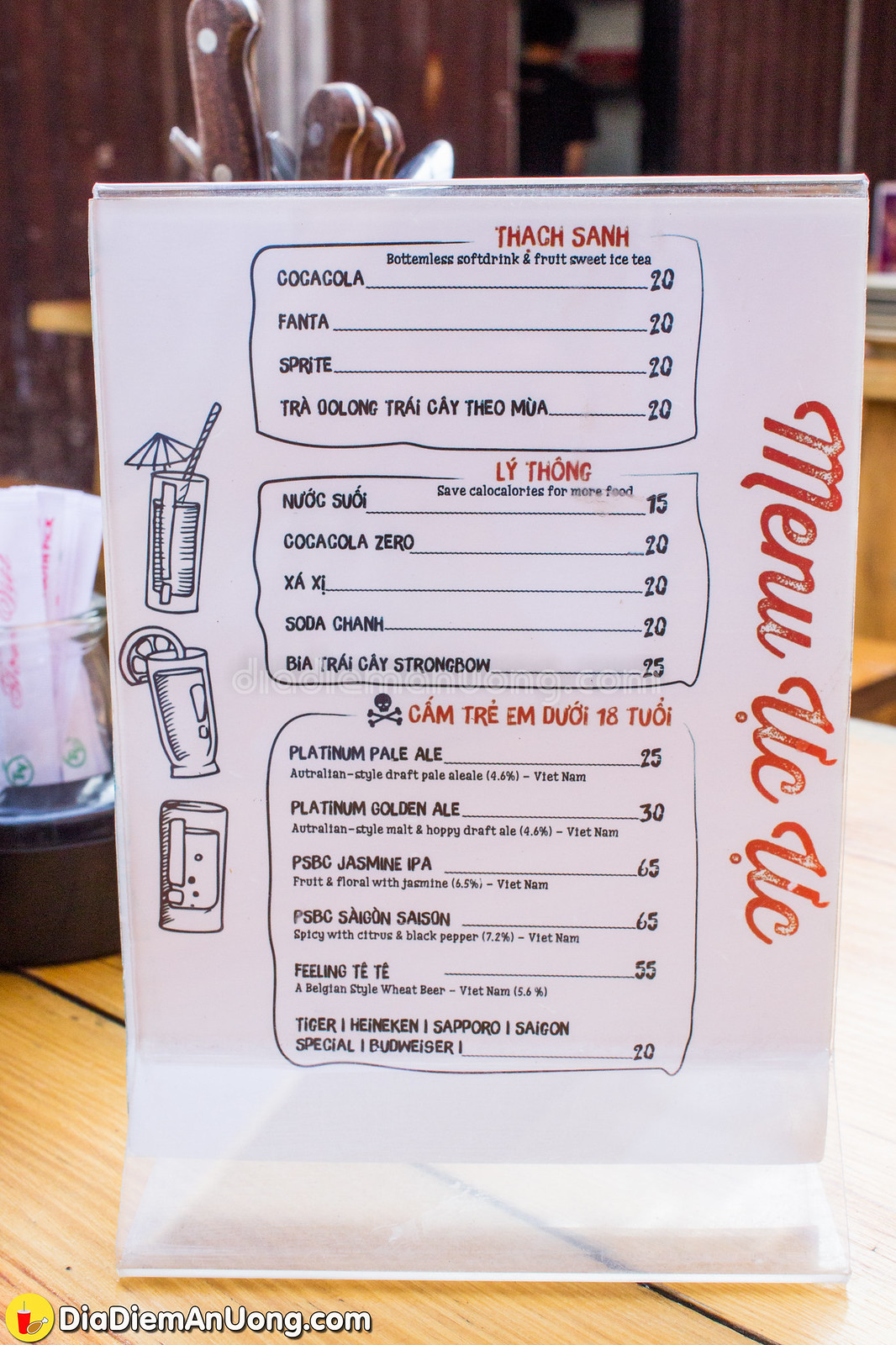This image showcases a stand-up menu from a Vietnamese restaurant, neatly placed in a transparent plastic holder that allows it to be easily displayed on a table. The menu features both Vietnamese and English text, catering to a diverse range of customers. At the top, it prominently displays the Vietnamese word "thac san," which suggests a category or special feature of the menu. Below, it lists items such as bottled soft drinks and fruit sweet iced tea, making it easier for non-Vietnamese speakers to understand the offerings.

The menu includes a section titled "lai thong," intriguingly captioned with "Save calories for more food," hinting at a lighter or health-conscious selection. Notably, some beverage names are provided in English, such as "Platinum Pale Ale," which is priced at 25 units, presumably in the local currency, Vietnamese Dong (VND).

At the bottom of the menu, the text "dia, dm, and uang.com" is visible, possibly referencing a website or additional information about the restaurant. The mention of "Vietnam" further confirms the cultural and geographic context of this establishment. Overall, this well-organized menu offers a glimpse into the Vietnamese dining experience, blending local and international elements for a comprehensive and approachable presentation.